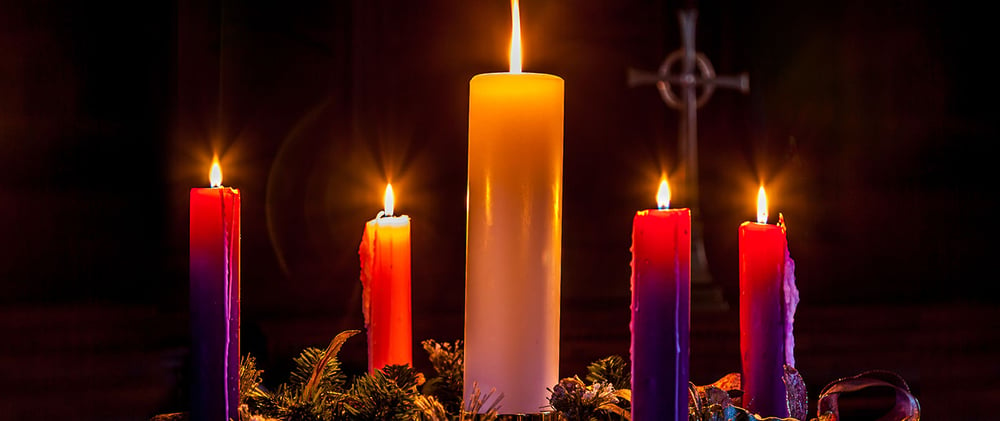This photograph captures a serene and reverent scene inside a church. Dominating the background, slightly right of center, stands a metal cross, framed by a circular element that is part of the cross's design. The scene is bathed in soft, warm light, likely emphasizing the spiritual atmosphere of the setting. In the foreground, five candles are prominently displayed. The central candle is a tall, white pillar, and it is flanked on either side by two shorter, standard candles. These side candles are deep red and exhibit a gradient ombre effect, shifting hues from red to purple, which may be enhanced by digital editing or the play of light and shadow in the image. All five candles are lit, their flames flickering gently. Surrounding the base of these candles are lush branches of what appears to be evergreen, adding a natural element to the setting. The image's colors are saturated and vibrant, likely digitally enhanced to accentuate the scene's visual impact.